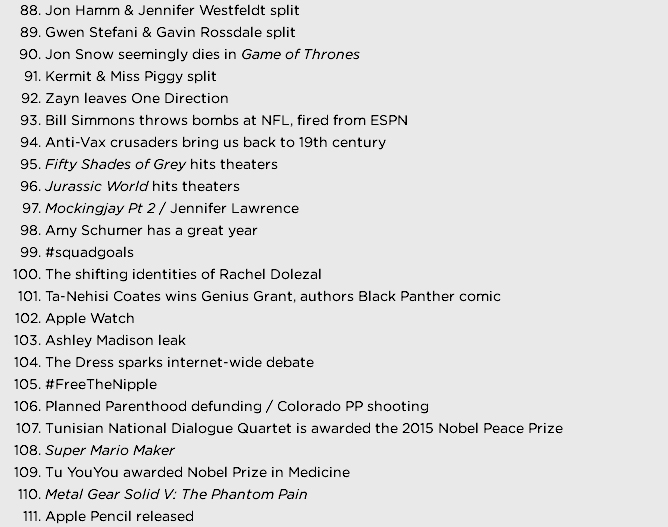A list of notable events and cultural moments is displayed in black text on a light gray background. The list is numbered from 88 to 111, covering a diverse range of topics from celebrity breakups to significant technological releases. Here is a detailed breakdown:

88. **Jon Hamm and Jennifer Wells-Fett split** - A breakup making headlines in celebrity news.
89. **Gwen Stefani and Gavin Rossdale split** - The end of a high-profile celebrity marriage.
90. **Jon Snow seemingly dies in Game of Thrones** - A shocking storyline development in the popular TV series.
91. **Kermit and Miss Piggy split** - The separation of the famous Muppet couple.
92. **Zayn leaves One Direction** - A major shift in the popular boy band.
93. **Bill Simmons throws bombs at NFL, fired from ESPN** - Controversial public statements by the sports commentator leading to his dismissal.
94. **Anti-vaxx crusaders bring us back to the 19th century** - A critical comment on the anti-vaccination movement.
95. **Fifty Shades of Grey hits theaters** - The release of the much-anticipated film adaptation.
96. **Jurassic World hits theaters** - The debut of the blockbuster movie.
97. **Mockingjay Part 2 / Jennifer Lawrence** - The final installment of the Hunger Games series featuring Jennifer Lawrence.
98. **Amy Schumer has a great year** - A notable rise in the comedian's career.
99. **#SquadGoals** - A popular social media trend emphasizing ideal friend groups.
100. **The shifting identities of Rachel Dolezal** - The controversy around Rachel Dolezal's racial identity.
101. **Ta-Nehisi Coates wins genius grant, authors Black Panther comic** - Recognition for the writer's contributions and his work on the Marvel comic.
102. **Apple Watch** - The release of Apple's smart wearable device.
103. **Ashley Madison leak** - A significant data breach revealing users of the infidelity-focused website.
104. **The dress sparks internet-wide debate** - The viral phenomenon over the color of a dress.
105. **#FreeTheNipple** - A social campaign advocating for gender equality and body positivity.
106. **Planned Parenthood defunding / Colorado PP shooting** - The contentious political and violent attacks on the organization.
107. **Tunisian National Dialogue Quartet is awarded the 2015 Nobel Peace Prize** - Recognition for promoting democracy in Tunisia.
108. **Super Mario Maker** - The release of the popular game allowing users to create their own Mario levels.
109. **Tu Youyou awarded Nobel Prize in Medicine** - Honoring the scientist's contributions to medicine.
110. **Metal Gear Solid V: The Phantom Pain** - The release of the critically acclaimed video game.
111. **Apple Pencil released** - The introduction of Apple's digital stylus.

This list encapsulates a range of milestones and cultural shifts within a specific timeframe, reflecting both popular culture and significant societal events.